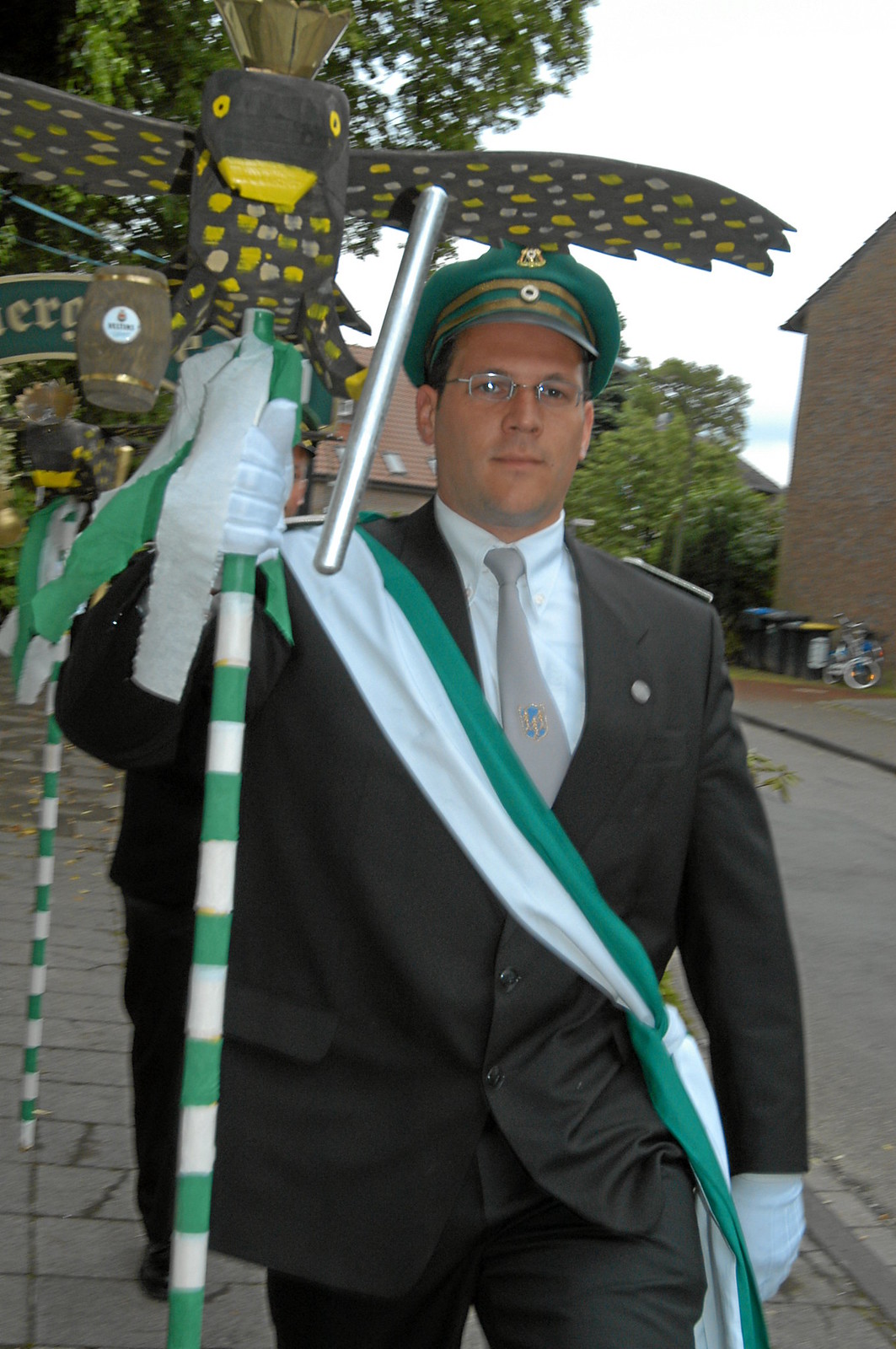This detailed photo captures a man who appears to be participating in a parade, dressed in a striking ensemble that blends formal and possibly military elements. He is wearing a dark suit paired with a white shirt and a gray tie, enhanced by white gloves. A distinctive green beret hat, adorned with buttons, sits atop his head, and he sports glasses. Draped across his chest is a green and white sash that extends from his right shoulder to his left hip, matching the colors of the green and white checkered pole he holds aloft in his right hand. The pole features an intricate, hard-to-identify decorative object on top, possibly resembling a large bird or insect, maybe even crafted from paper-mâché.

The setting is an outdoor urban area where several large buildings are visible to the right and behind the man. He walks along a brick sidewalk, and in addition to the buildings, the background reveals a variety of details, such as trees, a few bicycles, garbage cans, and a street sign. Another similar pole can be seen behind him, suggesting that he might be part of a larger group or float. The scene also includes other people and vehicles, adding to the ambiance of a bustling parade on what seems to be a cloudy day.